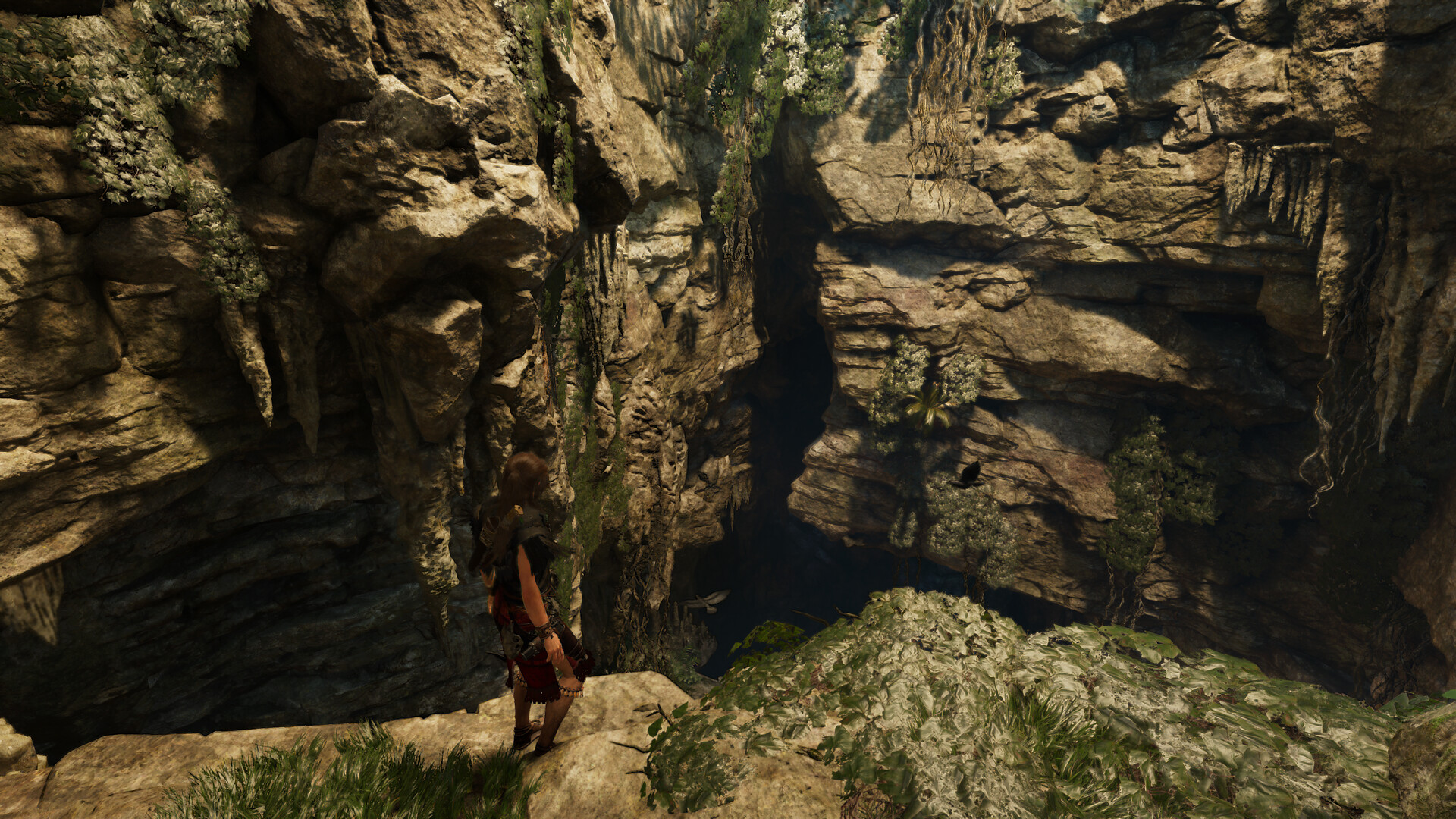The image is a vividly colorful depiction shown in landscape orientation. Dominating the foreground are numerous large boulders, atop which stands a slender, almost doll-like figure. This character, whose appearance hints at a computer-generated origin due to their unnaturally thin proportions and simplistic knee joints akin to those of a Barbie doll, is dressed in a brown and black outfit. Green patches of grass sporadically dot the rocky terrain. In front of the character lies an expansive wall of elongated rock slabs, their surfaces streaked with greenery. The figure gazes intently into a narrow crevice within the rock formation, seemingly contemplating how to navigate through the imposing barrier ahead.